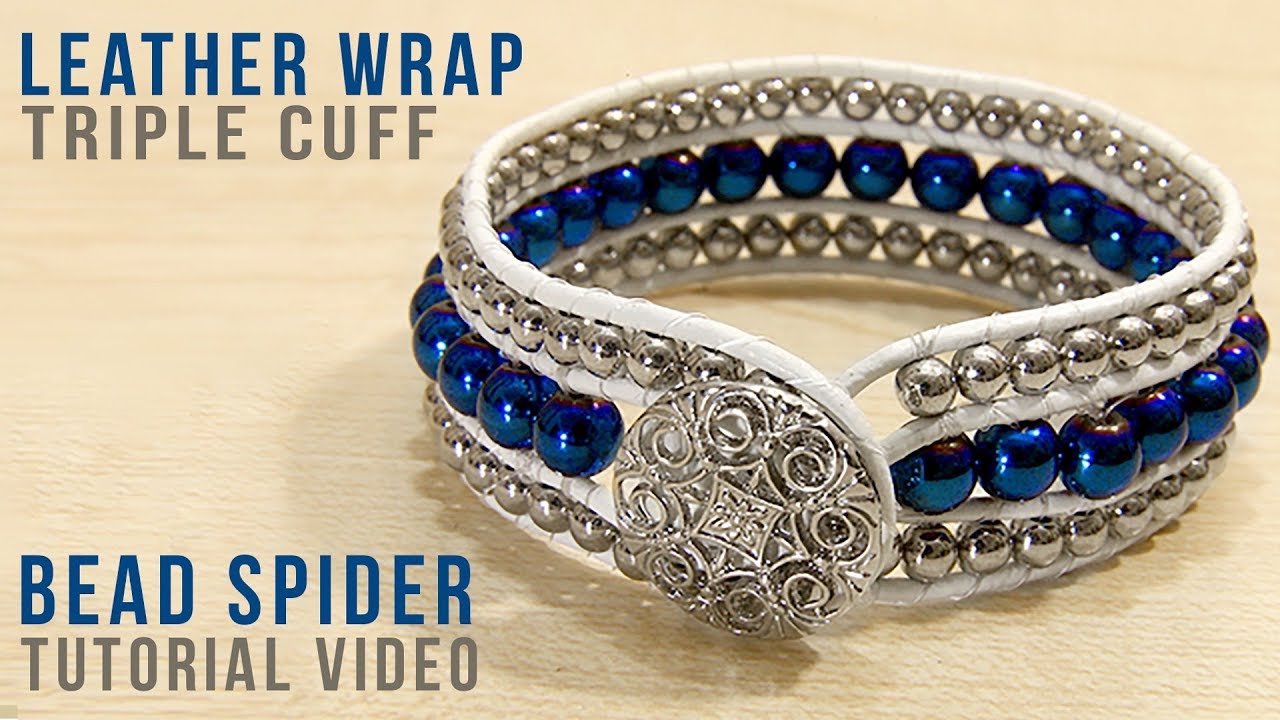In a clear and detailed image, the centerpiece is a striking white leather wrap bracelet, meticulously designed with alternating rows of silver beads and shiny blue pearls. This bracelet features multiple leather strands, intertwined with both the silver studs and vibrant blue beads, creating a layered and sophisticated look. A decorative, round metal clasp resembling a flower is prominently displayed at the center, adding an elegant focal point to the piece. 

The bracelet is displayed against a light wooden surface, enhancing its intricate details and craftsmanship. In the top left corner of the image, bold blue and gray text reads "LEATHER WRAP TRIPLE CUFF," and in the bottom right corner, it says "BEAD SPIDER TUTORIAL VIDEO," suggesting that this image is likely a thumbnail for a tutorial video. The pristine and reflective qualities of the blue and silver beads catch the light beautifully, making the bracelet appear even more luxurious.